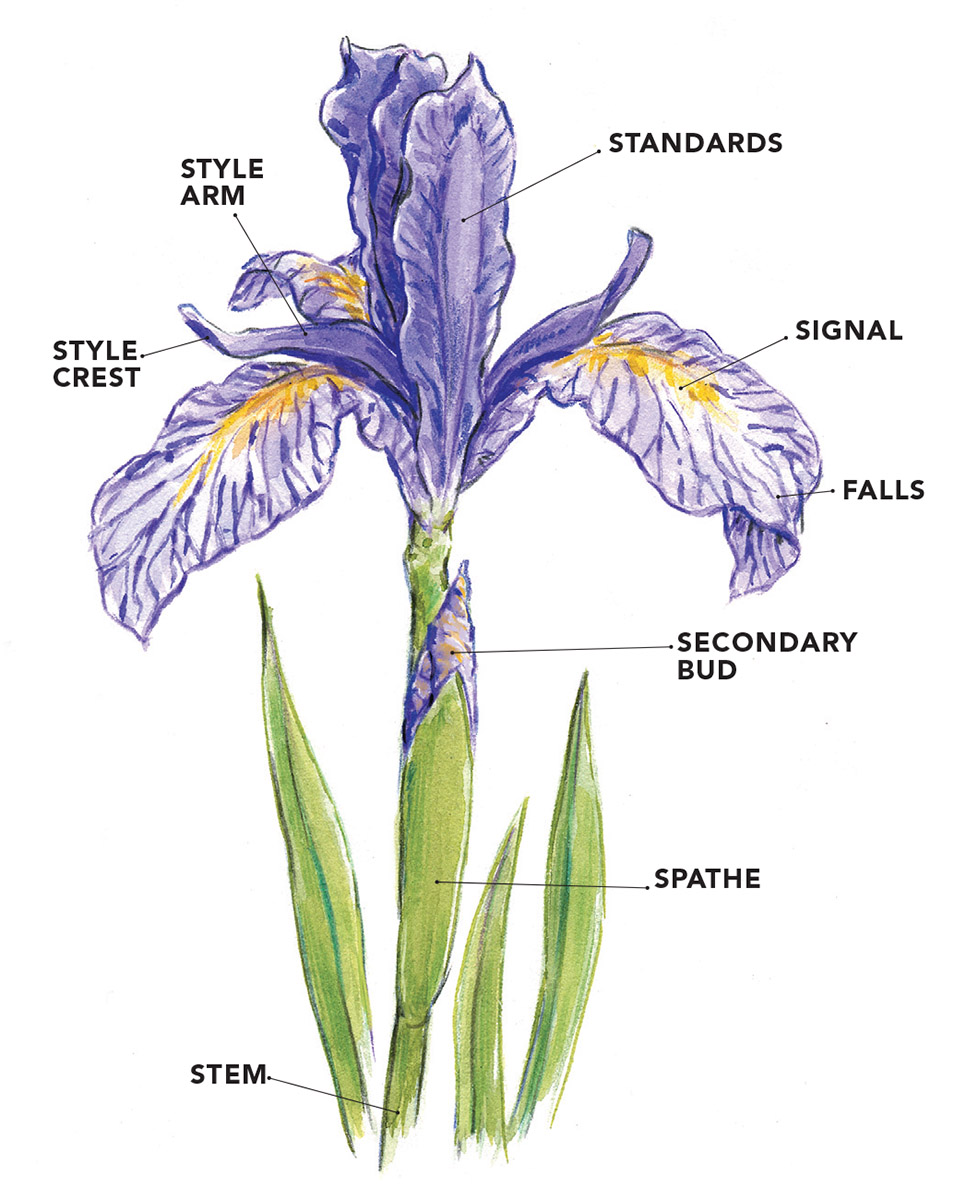This image is an illustrated diagram of a flowering plant on a white background. The diagram starts at the bottom with a green stem labeled "stem" in black text. This stem leads up to a leaf-like covering called the "spath," which may protect the flower. Moving upward, a secondary bud is indicated, suggesting it's not the main bloom but an additional one. 

At the flower section, various parts are meticulously labeled. The large flower has purple petals with some yellow and white details. The top left label "Style Crest" points to the end of the petals, and "Style Arm" points toward the inner parts of the flower. Labels for "Standards" are at the top part of the flower, while "Signal" points to the yellow sections and "Falls" to the white tips of the petals. The petals elegantly cascade over the sides, creating a visually appealing display. This detailed labeling provides a comprehensive understanding of the different parts of the flower.